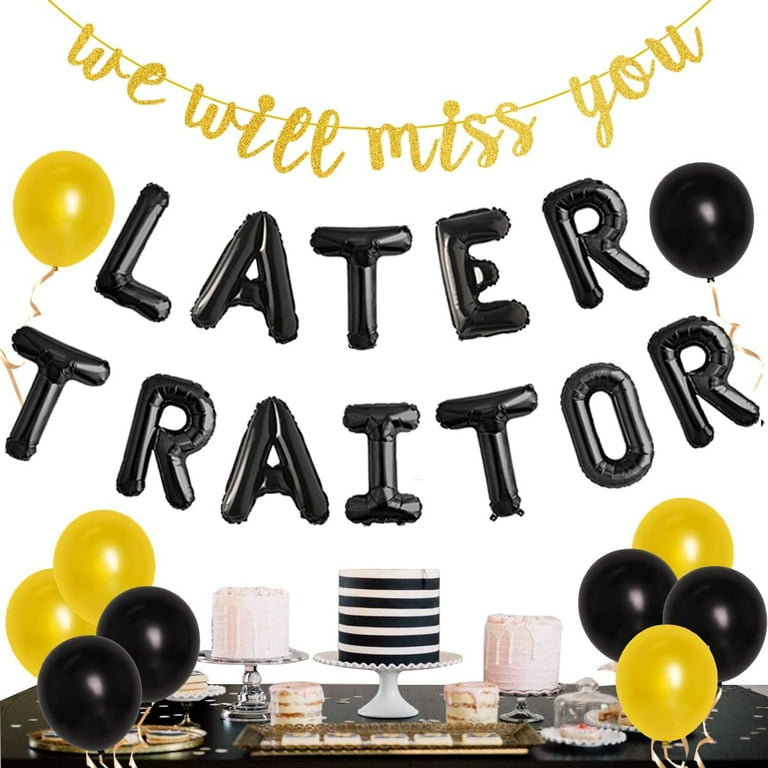The image depicts a meticulously arranged going-away party setup against a white background. At the top, small cursive gold letters strung from the wall spell out "we will miss you." Directly below, large balloon letters in black declare "later traitor," flanked by a yellow balloon on the left of the "L" and a black balloon on the right of the "R." Beneath this playful farewell message, the party scene is further decorated with clusters of balloons—on the left are two gold and two black balloons, and on the right, an identical set with an extra gold balloon at the bottom. The centerpiece is the table draped in a black tablecloth, sprinkled with white confetti. On the table stands a striking black-and-white striped cake on a cake stand, accompanied by two taller cakes in soft pink hues and two smaller white cakes. Additional small baked goods are neatly arranged under a glass cake dish, completing the festive display.